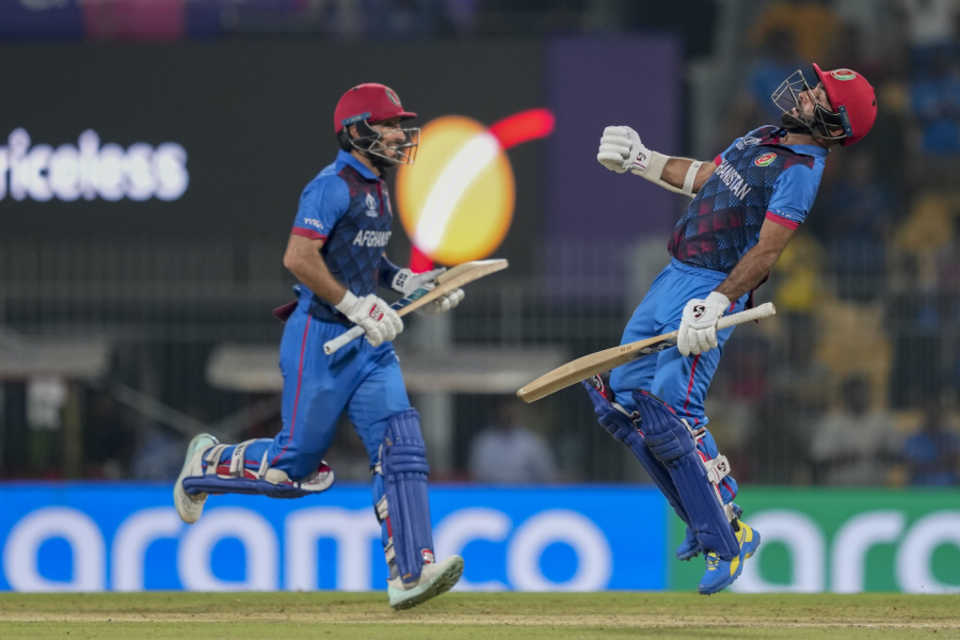The photograph captures a dynamic moment on a cricket field, featuring two cricket players in mid-action. Both athletes are donned in matching uniforms: blue pants, blue and red diamond-shaped jerseys, white gloves, red helmets, and blue shin guards. The player on the left is airborne, having jumped with a wooden mallet-like cricket bat in hand, expressing clear exultation. Facing him, the other player is in full stride, with one leg extended forward and the other kicked up behind, presumably heading toward the first player. The background showcases a blurry mix of spectators and advertising panels, including partially visible signs, one of which reads "Aramco" in large white letters. The playing field consists of patches of green grass and dirt, contributing to the overall sense of motion and excitement.